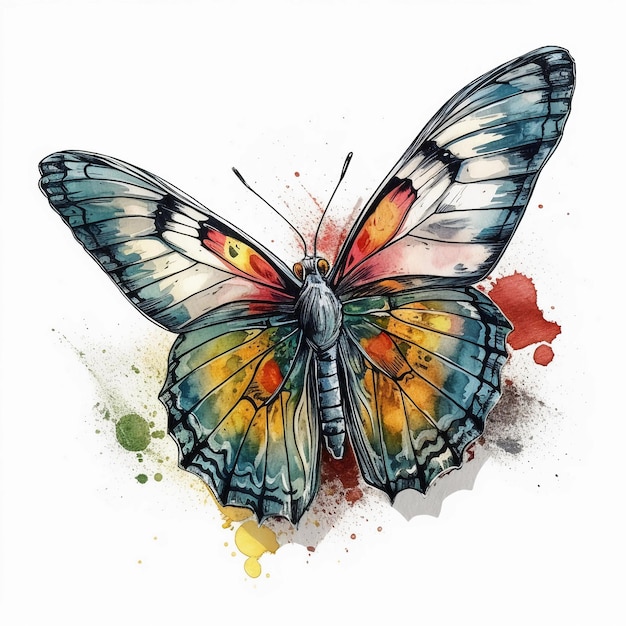This image features a striking piece of art, possibly digitally created or hand-painted, that showcases a large, cartoonish butterfly at its center. The butterfly, which dominates the white, frameless background, casts a shadow towards the bottom and right, suggesting a light source from above. The butterfly's body is bluish-gray, with a highly detailed, segmented tail and fur-like texture on its thorax. Its large, yellow eyes and black antennas give it an almost sinister look, as if it’s searching for something. The wings, which have a translucent appearance, are primarily bluish and white with intricate red and yellow detailing. Surrounding the butterfly are vibrant splotches of green, yellow, and red paint, adding to the artistic feel of the piece, as if the butterfly itself is a result of an expressive painting process.